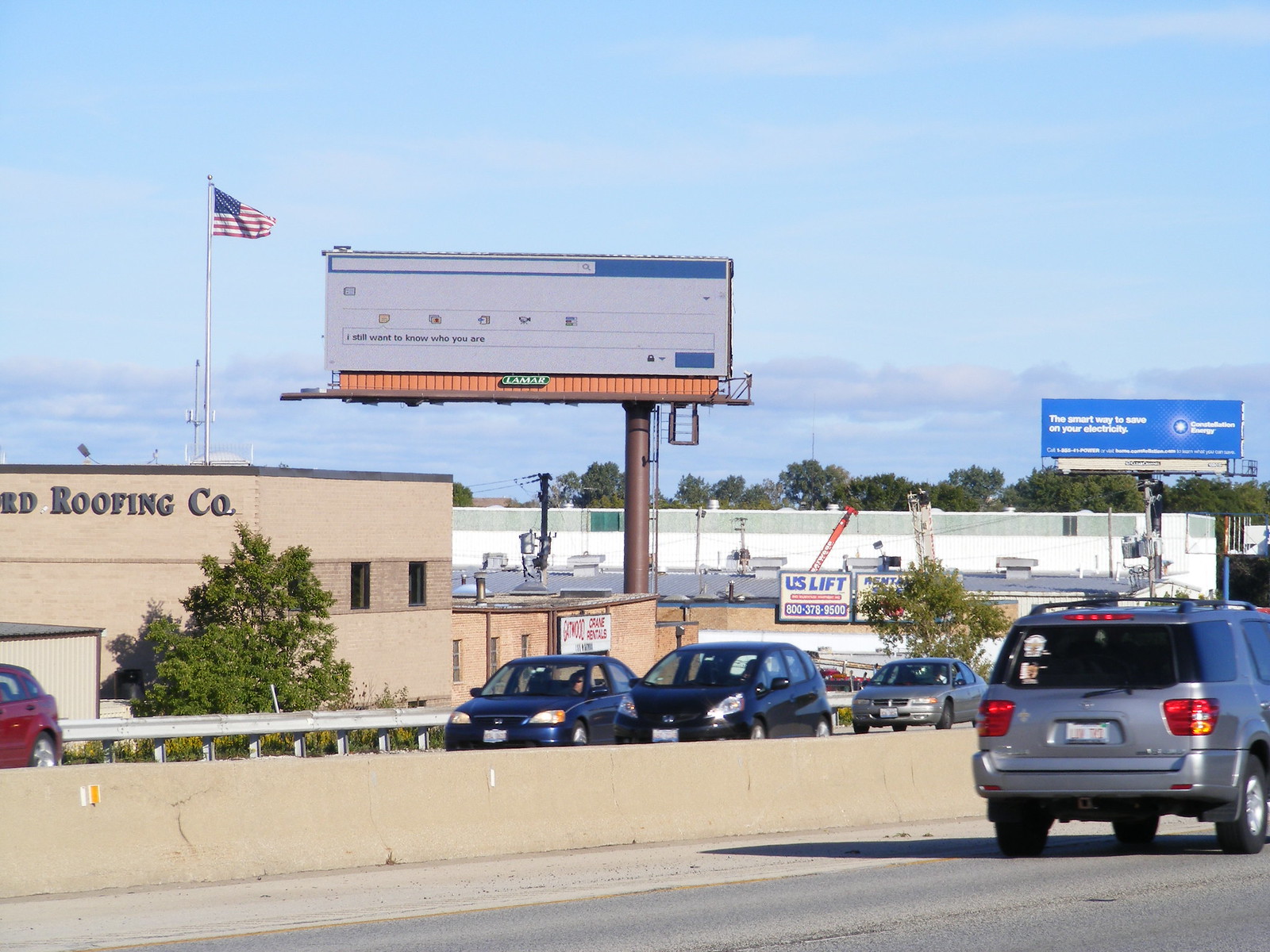The image depicts a freeway scene under a blue, partly cloudy sky. To the left, an American flag with red and white stripes is hoisted on a tall grey pole, soaring higher than the nearby billboard. The freeway is bustling with traffic, where vehicles travel in two lanes separated by a light grey cement barrier. In the closest lane, a grey SUV is moving from left to right, while on the opposite lane, several cars including a red one, two dark-colored vehicles, and a grey car move in the opposite direction. 

In the background, there are multiple industrial buildings, including a flat white structure with light grey siding. One of these buildings displays signage for a "Roofing Company," alongside another sign that reads "U.S. Lift," adorned with a blue box and a red box featuring white-lettered numbers. There is also a distinctive tree positioned in front of the Roofing Company building.

Further in the distance on the right side of the scene, two large billboards rise. The one to the left has a blue background with white letters, while the nearer billboard, featuring a partial web browser interface, enigmatically displays the text, "I still want to know who you are" in a search bar, suggesting a digital or startup advertisement. This composite scene captures the dynamic interplay of vehicular movement and the industrial urban landscape under an expansive sky.